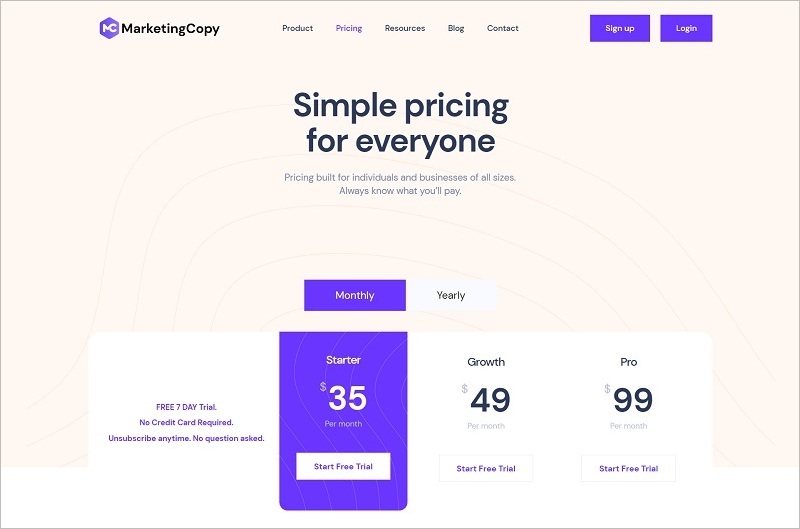This screenshot showcases the pricing page of a marketing website. At the top of the page, there are five navigation buttons in black for "Product," "Pricing," "Resources," "Blog," and "Contact." The "Pricing" button stands out in purple, indicating it is the currently active page. Additionally, there are "Sign Up" and "Log In" buttons in a purple or bluish box located at the top right.

The heading on the page reads "Simple Pricing for Everyone," followed by a subheading: "Pricing built for individuals and businesses of all sizes. Always know what you'll pay." Below the headings, there are two selectable options for the pricing plans: "Monthly" and "Yearly," with the "Monthly" option highlighted in blue.

The pricing structure includes three tiers:
1. **Starter**: $35 per month
2. **Growth**: $49 per month
3. **Pro**: $99 per month

Each plan offers a free seven-day trial with no credit card required and an easy, no-questions-asked cancellation policy. The page clearly emphasizes that users can start their free trial for any of the plans.

The overall design is user-friendly with clear call-to-action buttons and transparent pricing, ensuring visitors understand their options and the costs involved.